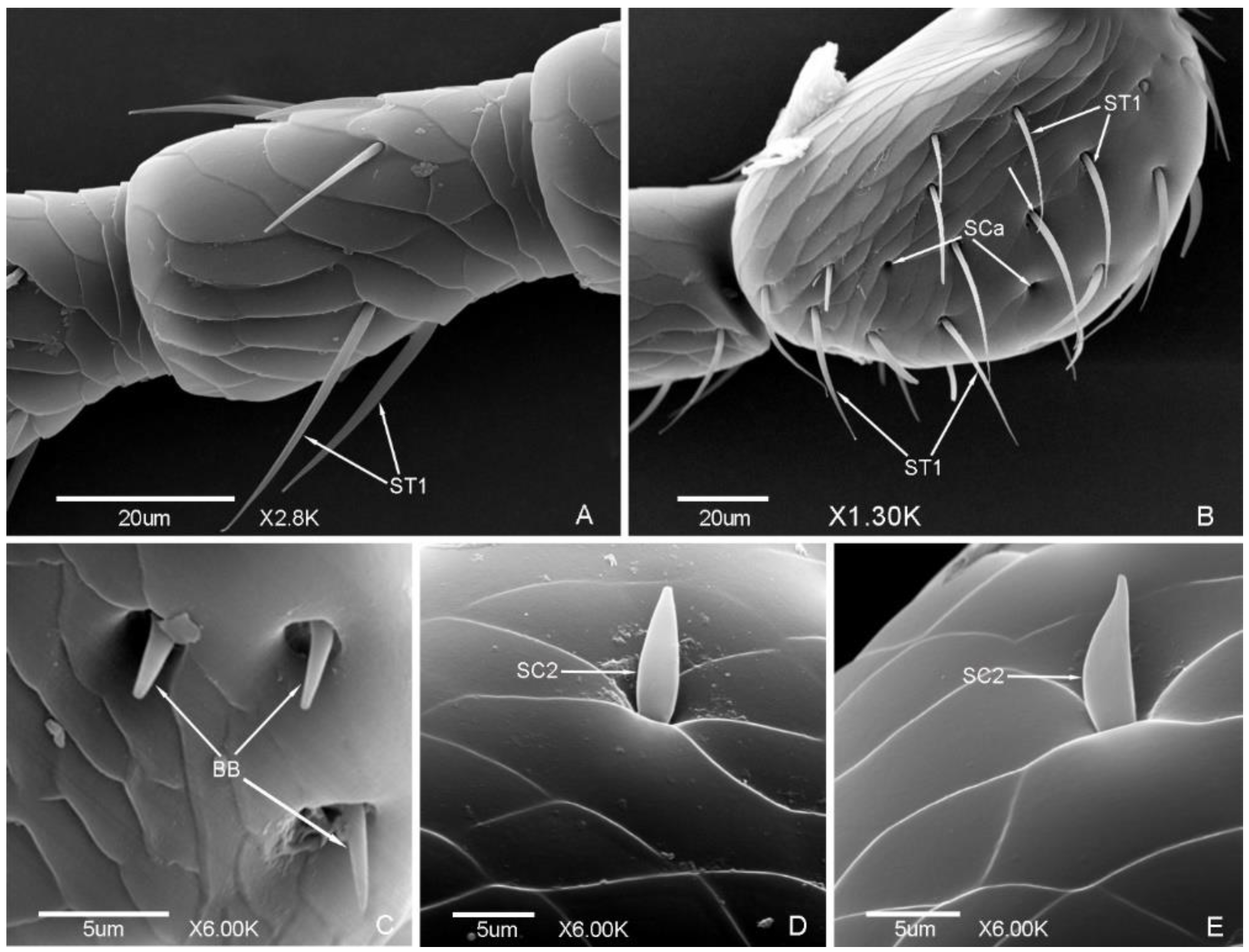This is a black-and-white microscopic image analysis displaying what appears to be a detailed close-up of an insect leg or a similar structure. The composition consists of five distinct micrographs, labeled A through E, situated in various corners and each zoomed in on different segments of the specimen. The images reveal intricate features, including flaky skin and spike-like hairs or follicles protruding from the surface.

Each micrograph contains white annotations and identification tags such as ST1 and SC2, with precise measurements indicated next to them, such as 20UM and 5UM, denoting microscopic scale. The images also include magnification details, represented as X 2.8K, X 1.30K, and X 6.00K, indicating various levels of zoom. The labeled sections are pointed out with arrows, directing attention to significant structures within the specimen. The overall visual presentation is a meticulous and structured microscopic examination, which could be useful for detailed scientific study.